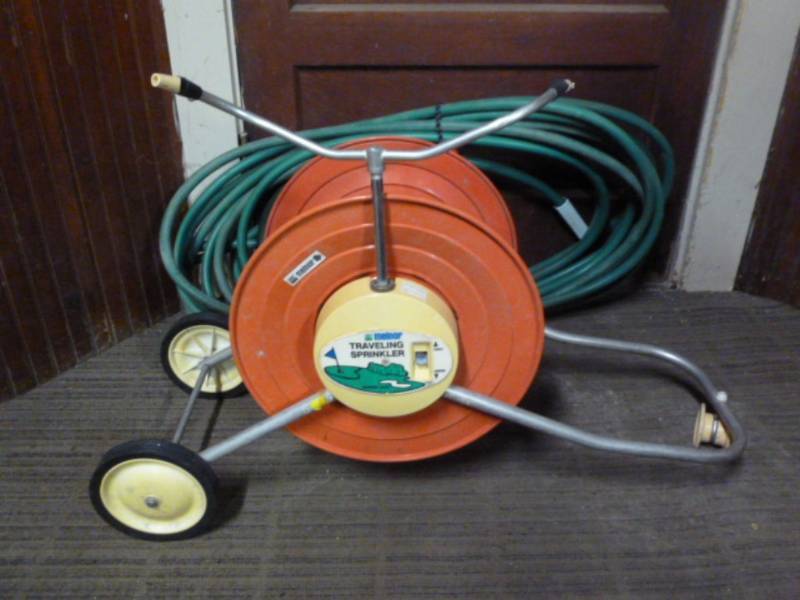This indoor photograph captures a vintage-style traveling sprinkler system, prominently positioned in the center. The orange, round spool of the sprinkler is affixed with two black wheels, which are detailed with yellowing edges, indicative of age. Attached to the central spool are metal bars that support the wheels. A distinct metal bar extends upward from the center of the sprinkler, dividing into two sections at the top, suggesting a mechanism that spins to distribute water as it moves slowly across a lawn. The label on the spool reads "traveling sprinkler" and features an image of a golf course, adding to its vintage charm. A silver handle on the side and another on top, resembling a bike handle, offer ease of mobility. This sprinkler system is situated on a gray carpeted area, flanked by walls of long vertical dark wood planks and a brown door. Behind it, a green garden hose is neatly coiled, further indicating the setting's indoor nature.